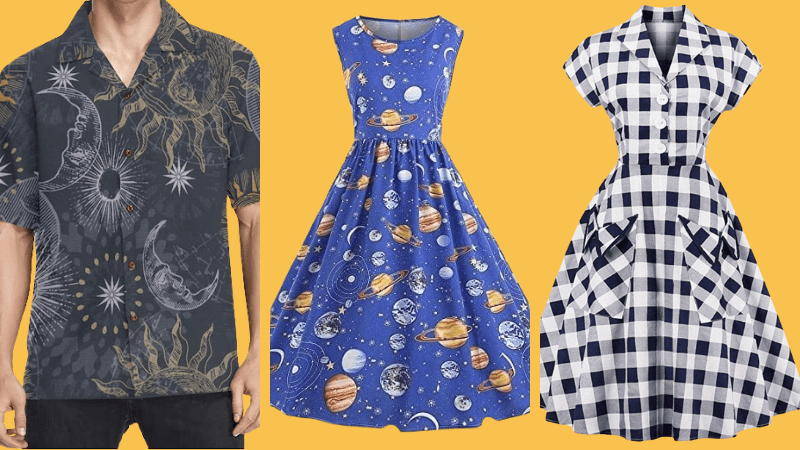The photograph features three distinct subjects set against a muted orange background. On the far left, a headless male figure wears a dark short-sleeve button-up shirt adorned with whimsical patterns of the moon, sun, and stars, paired with dark jeans. In the center, there is a sleeveless dress with a scoop neck, predominantly blue with an imaginative print of planets and stars, evoking a celestial theme. On the right, a checkered dress with a black and white tablecloth pattern hangs empty. The dress features short sleeves, a full skirt, and three buttons down the front, with large pockets. The overall composition highlights the three items of clothing in a visually striking manner.